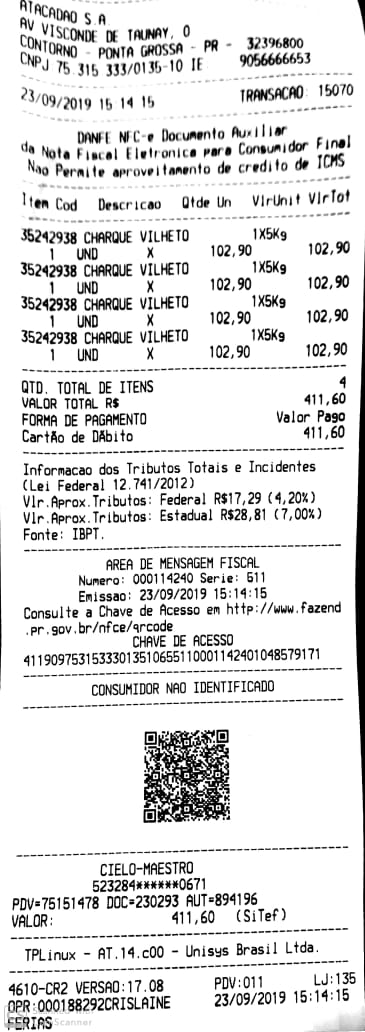This is an image of a photocopied receipt featuring an extensive and crisp amount of detail. The receipt itself occupies most of the image, with a small black strip visible along the right edge, likely an artifact from the photocopying process. At the top of the receipt, there's text in a foreign language, specifically displaying "AIACADAO S O," which appears to be part of the store or company's name. The total amount on the receipt is $411.60. It indicates the purchase of four identical items, each priced at $102.90. Additionally, a QR code is located at the bottom of the receipt, possibly for easy access to digital details or for scanning purposes.